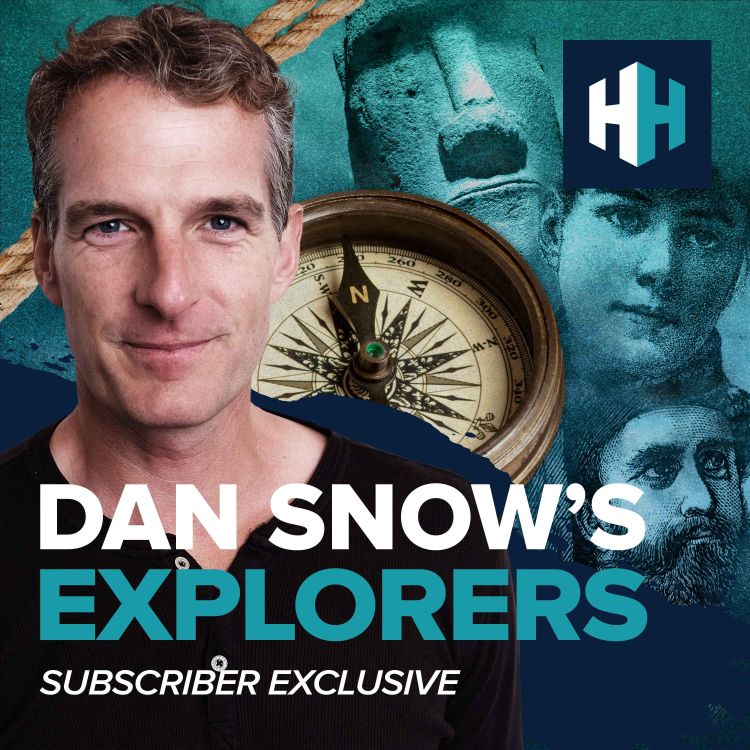In this advertisement, a promotion for "Dan Snow's Explorers," we see a detailed and intriguing layout designed to attract subscribers. Dominating the left side of the image is Dan Snow, a Caucasian man with brown hair accented by gray streaks. He wears a subtle smile with his mouth closed. Below his portrait, in bold white and blue text, is the title "Dan Snow's Explorers," followed by "Subscriber Exclusive" in white letters. 

The background showcases a compass pointing north, symbolizing exploration and discovery. Surrounding the compass are various historical elements: intricately coiled Nautilus ropes, an ancient artifact resembling a tiki statue, and images of two historic figures, one male and one female. On the left side is a glimpse of Stonehenge, adding a touch of mystery and prominence to the theme of exploration. 

In the top right corner, the emblem of the History Channel is displayed in a dark blue box, featuring the distinctive white and light blue interlocking "H" letters. This combination of visual and textual elements builds a compelling invitation to viewers, emphasizing exclusive content available to subscribers.